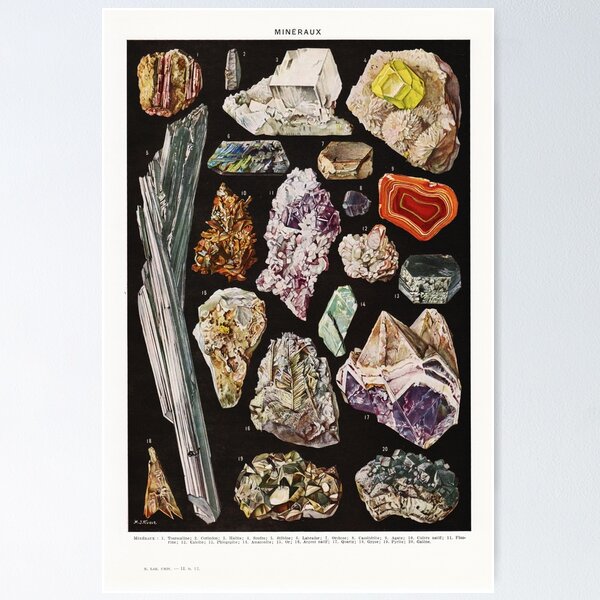The image depicts a detailed scientific chart resembling a page out of a book or a magazine, showcasing various types of minerals and quartz. At the top of the chart, the word "Minéraf" (M-I-N-E-R-A-U-X) is prominently displayed in black text. The chart features around 15 different examples of quartz, meticulously illustrated to highlight their distinct crystalline structures. Noteworthy specimens include a brown quartz situated in the top left corner, adjacent to a clear quartz embedded in a larger rock. Further along, a tan rock with a yellow quartz crystal in it can be observed. The chart also includes a diverse range of crystal colors like purple, red, and yellow, all set against a striking black background. A white border frames the poster, with the names of the minerals written in small print along the bottom. Additionally, there is a distinctive long mineral sample running almost the full length of the left side, and in the upper right section, a mineral that appears to be gemstone-bearing. This well-organized display of mineral and quartz samples serves as an informative diagram, typical of scientific publications.